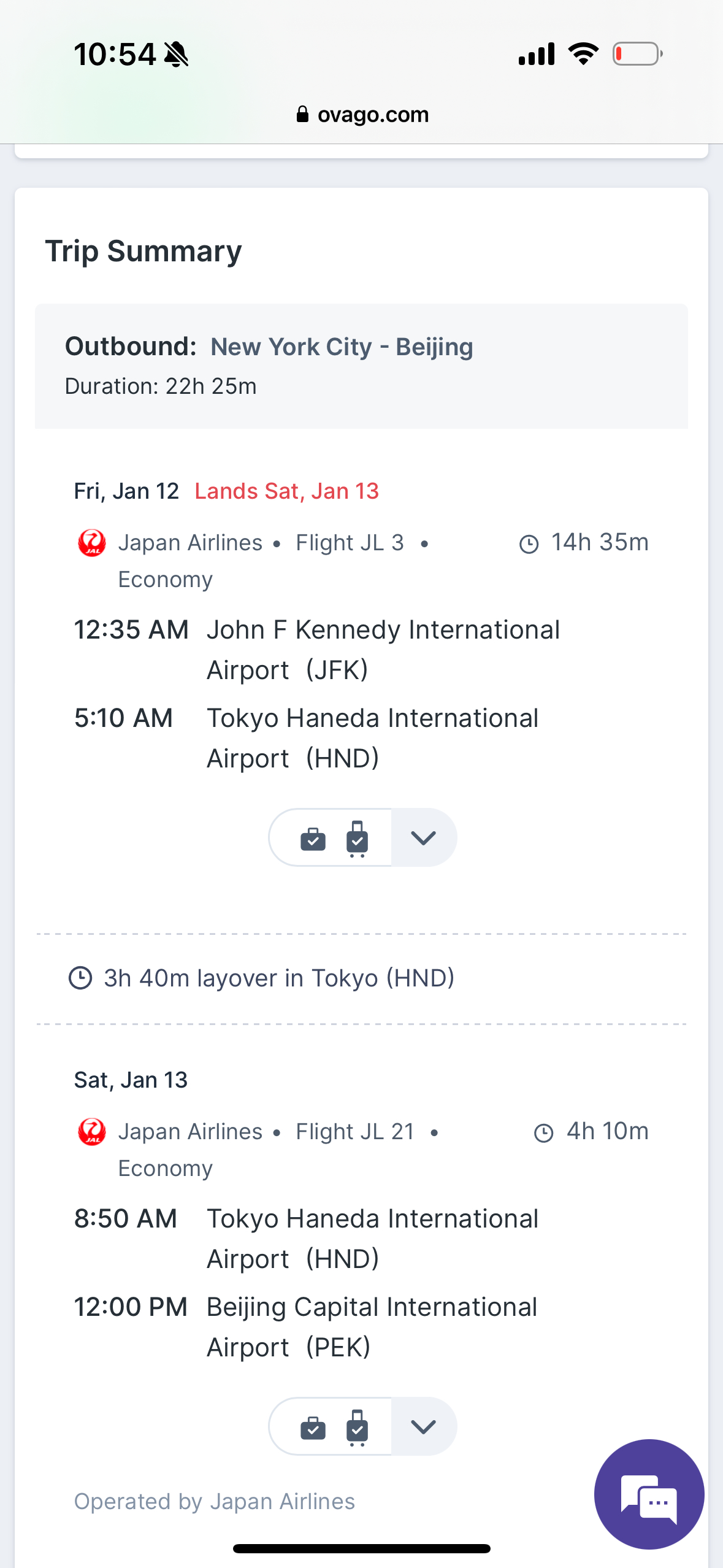The screenshot appears to be from a mobile phone displaying a detailed trip summary on the website "ovago.com." At the top of the screen, a lock icon indicates a secure connection. The time is displayed as 10:54, and the status bar shows full Wi-Fi reception and cellular connection but a nearly empty battery, indicated by a red battery icon.

The main content of the screen details a trip itinerary:

- **Outbound Flight**: From New York City to Beijing.
  - **Total Duration**: 22 hours and 25 minutes.
  - **Departure**: Friday, January 12th.
  - **Arrival**: Saturday, January 13th.
  - **First Leg**: 
    - **Flight**: Japan Airlines JL3.
    - **Duration**: 14 hours and 35 minutes, Economy Class.
    - **Departure Time**: 12:35 a.m. from John F. Kennedy International Airport (JFK).
    - **Arrival Time**: 5:10 a.m. at Tokyo Haneda International Airport (HND).
    - **Icons**: Luggage symbols are present, likely indicating checked baggage details.
  - **Layover**: 
    - **Location**: Tokyo Haneda International Airport (HND).
    - **Duration**: 3 hours and 40 minutes.
  - **Second Leg**:
    - **Flight**: Japan Airlines JL21.
    - **Duration**: 4 hours and 10 minutes, Economy Class.
    - **Departure Time**: 8:50 a.m. from Tokyo Haneda International Airport (HND).
    - **Arrival Time**: 12:00 p.m. at Beijing Capital International Airport (PEK), noted in parentheses.

At the bottom of the screen, there is a purple chat button with two white chat bubble icons, suggesting customer support or live chat assistance.

The visual elements and detailed text provide a comprehensive overview of the travel itinerary from New York City to Beijing with a layover in Tokyo, operated by Japan Airlines.